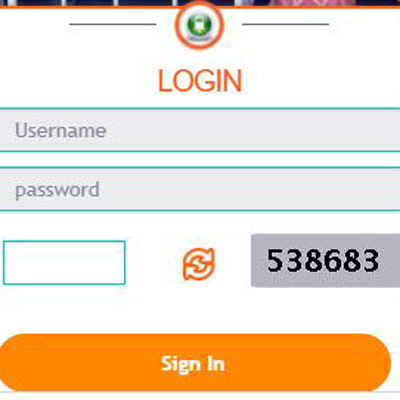The image features a close-up view of a login page, so close that the top part of the window is slightly cropped, obscuring the context of what one would be logging into. The login interface appears to be a pop-up window, but the tight framing makes it seem like the primary window. 

At the very top of the image, a thin strip of the background is visible, which appears to be predominantly black with several white lines and a touch of pink. The login window itself is outlined by a thin orange line. Centrally placed at the top of this window is a circular emblem with an orange border and a white center, housing a green sphere in the middle, which contains a smaller white object at its core.

Directly below this emblem, the word "LOGIN" is prominently displayed in uppercase orange letters, centered along the horizontal axis. Following this heading are the input fields for the username and password, neatly aligned to allow users to enter their credentials. This detailed close-up emphasizes the design elements and layout of the login interface while capturing a glimpse of the surrounding environment.